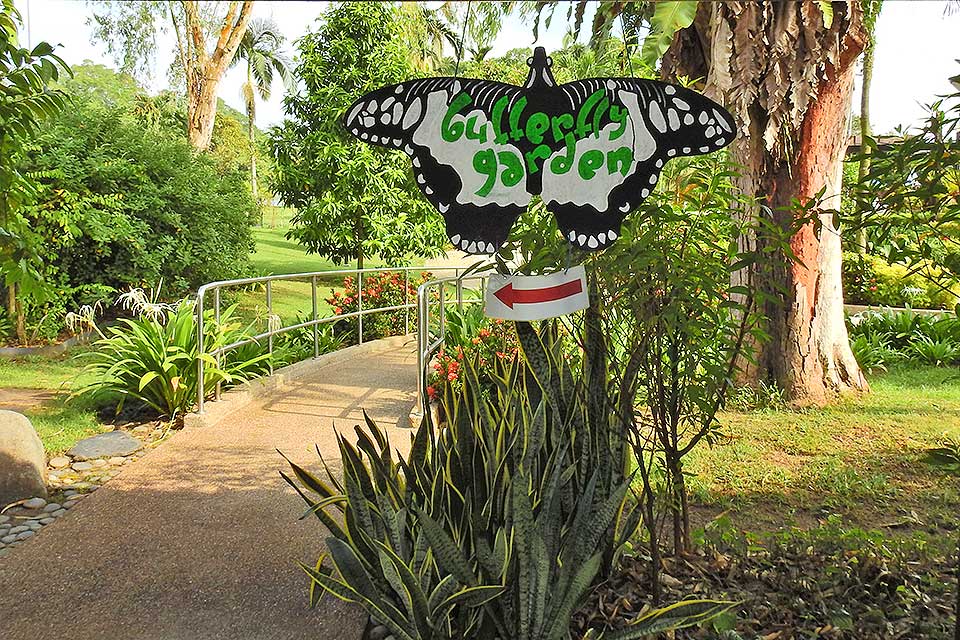The photograph depicts the entrance to a Butterfly Garden, featuring a large, butterfly-shaped sign with green lettering that reads "Butterfly Garden" and a red arrow pointing to the left. This sign is strategically placed among lush, dark green, pointed plants and is complemented by a well-defined walkway with silver railings on either side. The garden exudes a tropical ambiance, showcased by an array of trees, bushes, and wild plants flourishing in the surrounding grassy area. Notably, there is a sizable rock purposefully positioned on the left side, and one tree appears to be damaged, possibly by lightning. The background features additional large trees and bushes, further accentuating the natural, verdant setting.